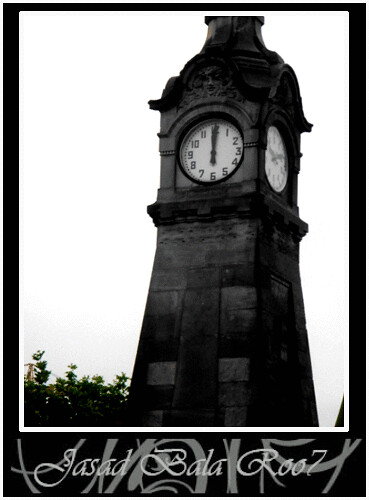The image features a black and white photo of a large architectural structure, prominently displaying a clock at the top. The clock face directed towards the viewer shows both hands precisely at the 12 o'clock mark. Intriguingly, there is a second clock face on the opposite side of the building, with its hands pointing in different directions, adding a layer of mystery to the scene. The entire picture is set within a decorative black frame, beneath which, in a cursive font, are the letters "j a s a d b a l a r o o" followed by the number seven. Surrounding the black frame, there is an additional white border which completes the presentation of the photo.